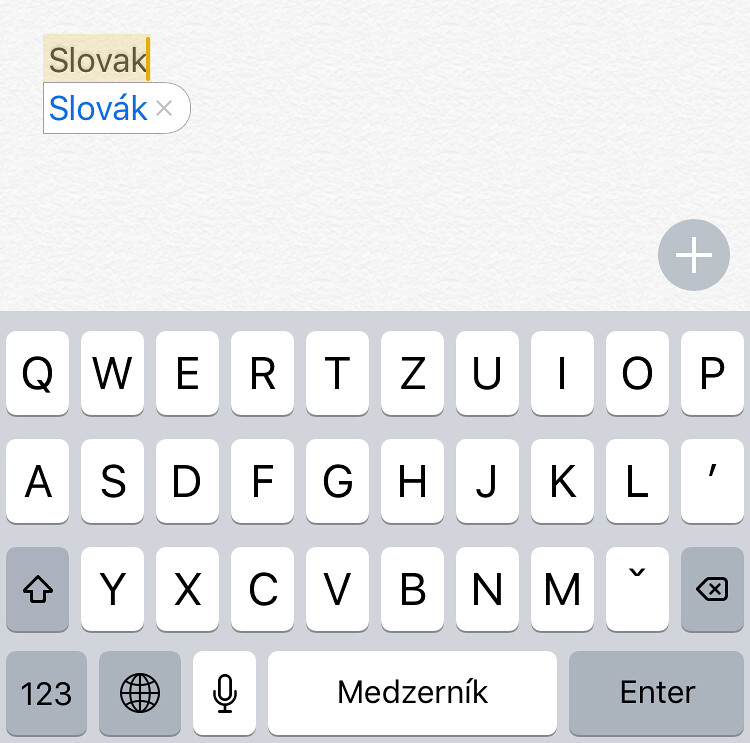This screenshot captures a cell phone's digital keyboard in action. Dominating the screen is the keyboard, which features a gray background, white keys, and black letters. Notably, the keys include common elements such as a gray "Enter" button, a gray globe icon, and a gray "123" key for numeric input, along with gray arrow keys. Central to the keyboard layout is a white space bar inscribed with the term "MEDZIRNIK" in black.

At the top of the image, the text box displays the word "SLOVAK" in black text on a yellow background in the upper left corner. Directly beneath it is an autocorrect suggestion: the same word but with an accented 'A' (S-L-O-V-A´-K), rendered in blue text against a white background, with an "X" icon indicating the option to dismiss the suggestion. Additionally, a white circular icon with a plus sign sits on the right, slightly below the midpoint, suggesting an option to add a contact or input. The keyboard layout includes all standard keys, like 'QWERTY', 'ASDF', and an 'Up' arrow, making it a familiar digital keyboard interface at a glance, but the presence of foreign words indicates that it is configured in a different language.